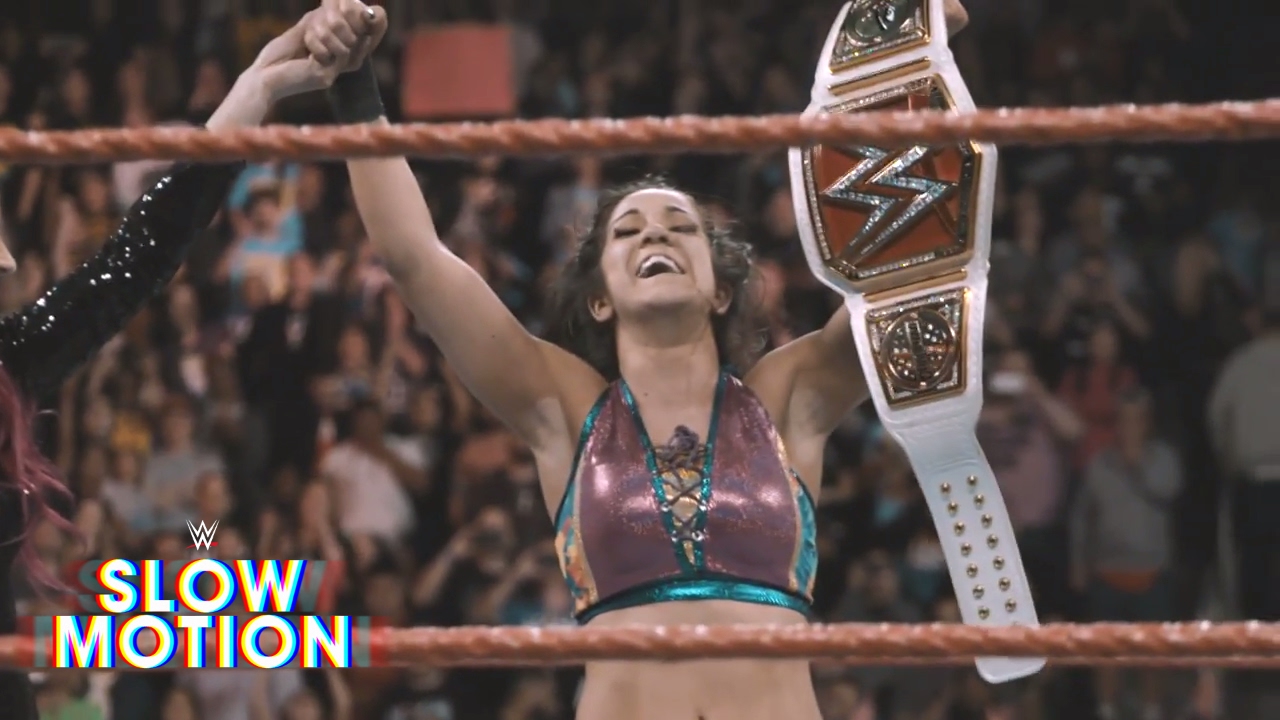In this captivating image from a WWE event, we see Bayley in the wrestling ring immediately after a victorious match. She is beaming proudly, her bright smile revealing teeth, as she holds the WWE Women's Championship belt aloft in one hand. The championship belt, predominantly white with a striking red center featuring the iconic silver and red "W", is a testament to her triumph. Bayley is adorned in a vibrant short sports bra vest that is predominantly purple, accented with green on the sides and straps, likely paired with matching bottoms. The scene is heightened by the presence of another woman, partially visible beside her, believed to be Becky Lynch, dressed in black leather attire. This celebratory moment is captured with the WWE logo and the word "SLOW MOTION" in white lettering on the bottom left corner, adding a dramatic flair to her moment of victory as fans behind her cheer in jubilation.